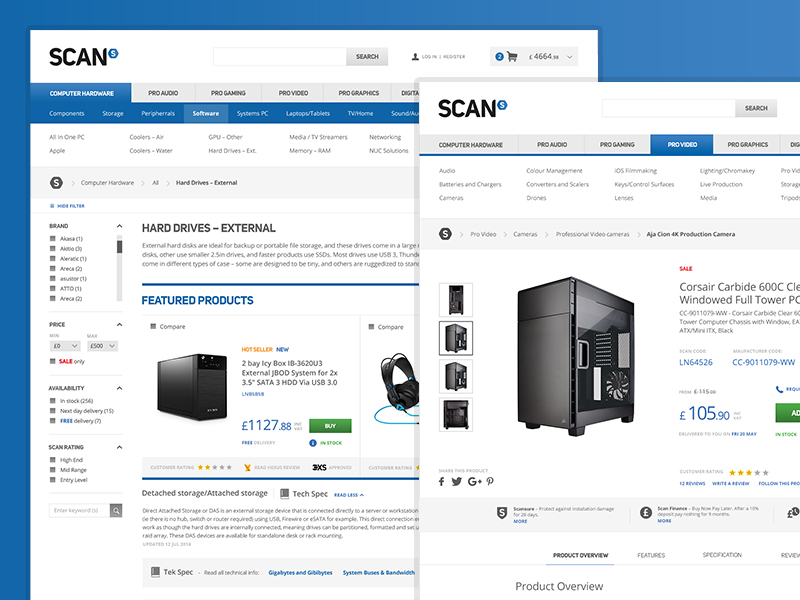**Caption:**
The image captures a website scan displaying two open tabs, side by side. The tab on the right prominently features a Corsair GearBuddy 600C window full-tower PC case, priced at £105.90. The other tab, partially visible in the background, appears to show various external hard drives. Notably, the highlighted product in the back tab is priced at £1,127.88, suggesting a high-end item. Both prices are displayed in pounds (£). Additionally, the website features the 'SCAN' logo in all uppercase letters, accompanied by a small currency symbol. This setup indicates that the viewer was likely comparing different tech products, possibly for research or purchasing purposes.